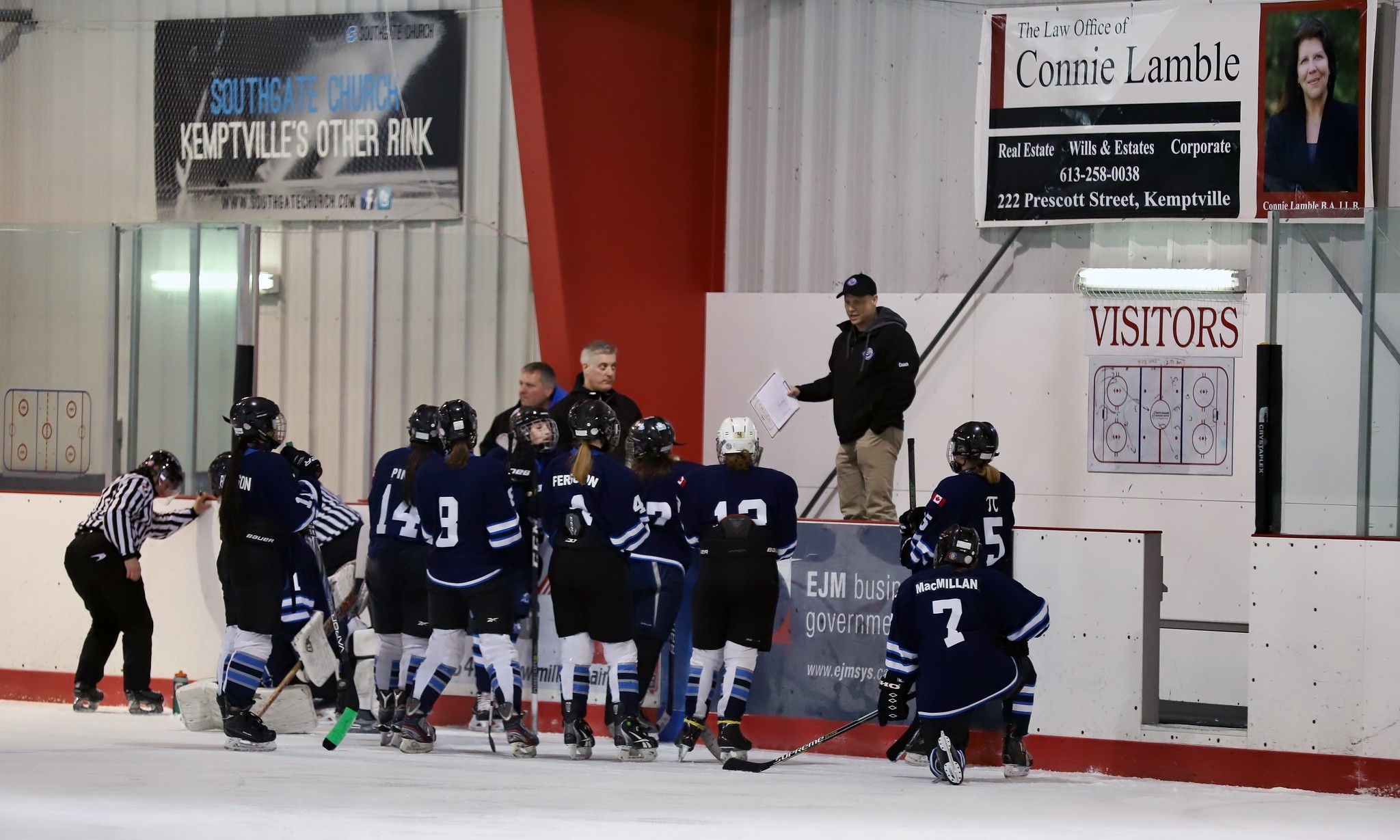The image depicts an indoor ice hockey rink featuring a team of hockey players in dark blue jerseys with white numbers on their backs, black helmets, and one player wearing a white helmet. The players, all female, are gathered at the edge of the rink, fixated on their coach who is standing elevated, possibly on a podium or bench, wearing a black coat and baseball cap and holding a clipboard or whiteboard in his right hand. Nearby, two referees in black and white shirts with black helmets stand on the far left. 

The backdrop includes various advertisements plastered on the walls of the rink. In the upper right corner, there's a banner for the "Law Office of Connie Lambie" detailing services in real estate, Wilson Estates, and corporate law, along with a phone number and address: 613-258-0038, 222 Prescott Street, Kemptville. In the upper left corner, another banner reads "Southgate Church," highlighting "Kemptville's other rink" in white text on a blue background. Additionally, there are advertisements for EJM, a business/government entity, in red, white, and blue colors along the wall. Above the players' heads to the right of the coach is the word "VISITORS" in red letters, accompanied by a diagram of the hockey rink from a bird's-eye view.

Overall, the rink is bustling with activity, the ice and surrounding boards gleaming under bright overhead lights, framed by the white walls of the building.